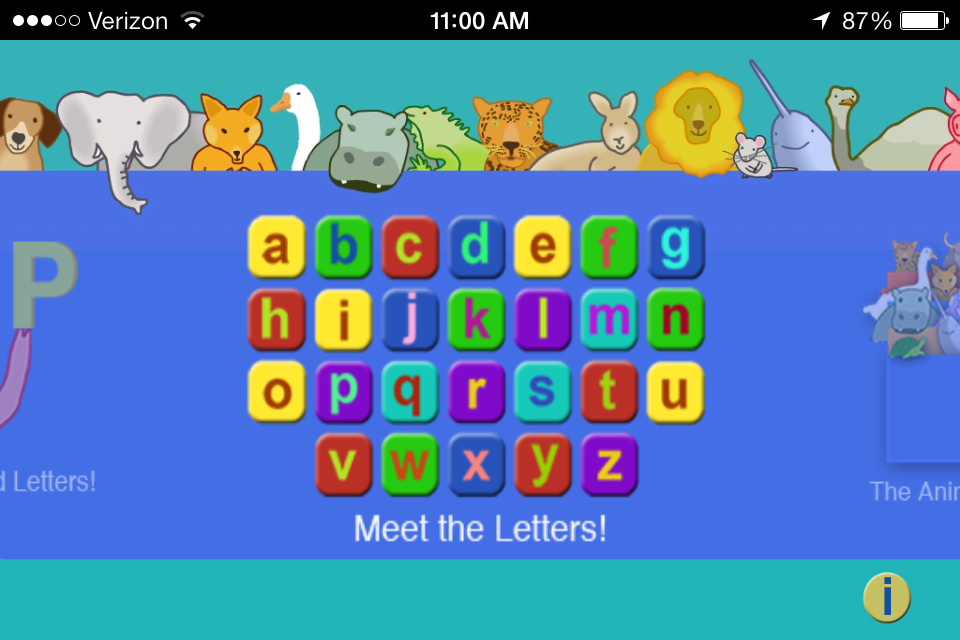The screen capture depicts a children's video game on a smartphone, with "Verizon" displayed in the top left corner. The screen indicates it is the third page of a five-page sequence, as shown by three illuminated white dots and two unlit black dots. The time shown is 11:00 AM, positioned centrally in white text. The battery level is at 87%.

The main area of the screen is dominated by a large teal background showcasing a variety of animals: a dog, an elephant, a fox, a duck, a hippo, a lizard, a jaguar, a kangaroo, a lion, a mouse, a narwhal, an ostrich, and possibly a pig.

Below the animal illustrations, there is a row of colored boxes, each containing a letter of the alphabet. The text "Meet the Letters" is prominently displayed in white beneath these boxes. Further down, part of the teal background is visible again, accompanied by a yellow information icon featuring a blue letter "i" in the bottom right corner.

Additional animals or the same ones seem to be in a blue box on the right side of the screen, interspersed with the alphabet letters. The far left of the screen includes more text and possibly more animal illustrations, though this section is partially cut off.